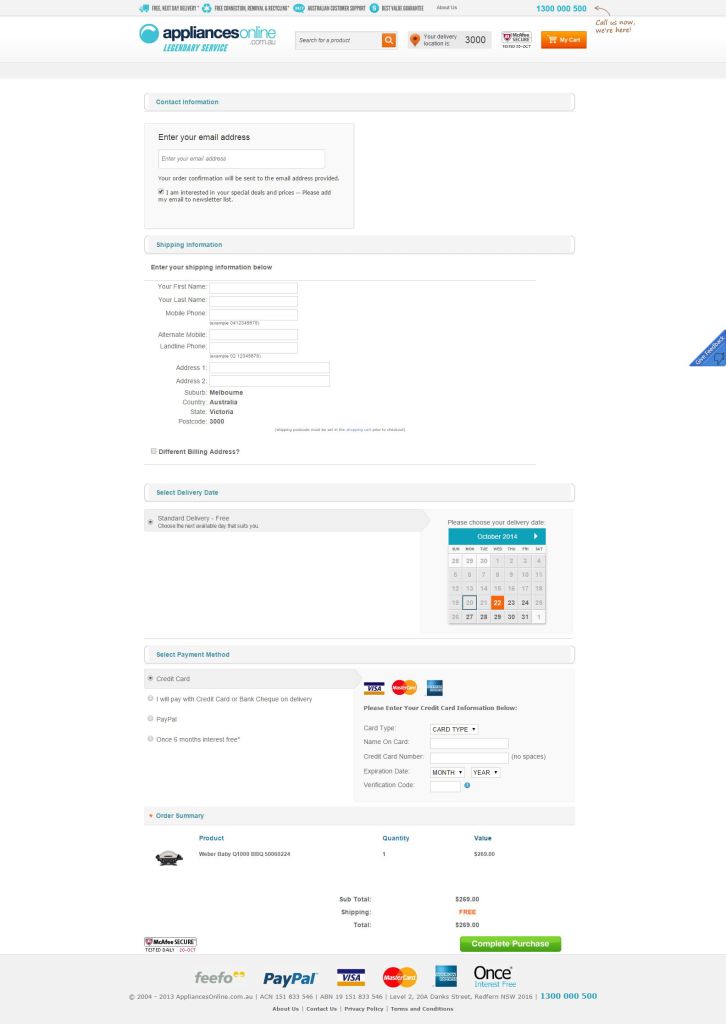This small screenshot from the Appliances Online website showcases several key elements despite its size. The logo is prominently displayed on the top left corner, featuring a light blue circle with dark blue text for "Appliances" and light blue text for "Online". Directly to the right, there is a search bar highlighted by an orange search button, followed by a location button, a security notice, and a "My Cart" button for accessing the shopping cart.

Navigating downward, the website appears to have four distinct rows of information. The first row includes some unclear text, which might be related to purchase or billing/shipping details. The second row contains a section dedicated to calendar functionalities. In the third row, payment options are displayed, supporting Visa, MasterCard, and American Express.

Lastly, additional product information is provided in the fourth row, which features various text input fields for entering personal details such as first name, last name, phone number, and address information. In the top right-hand corner of the screenshot, a company phone number is visible, ensuring customers can easily contact support if needed. The entire webpage is set against a clean, white background, enhancing readability and navigation.